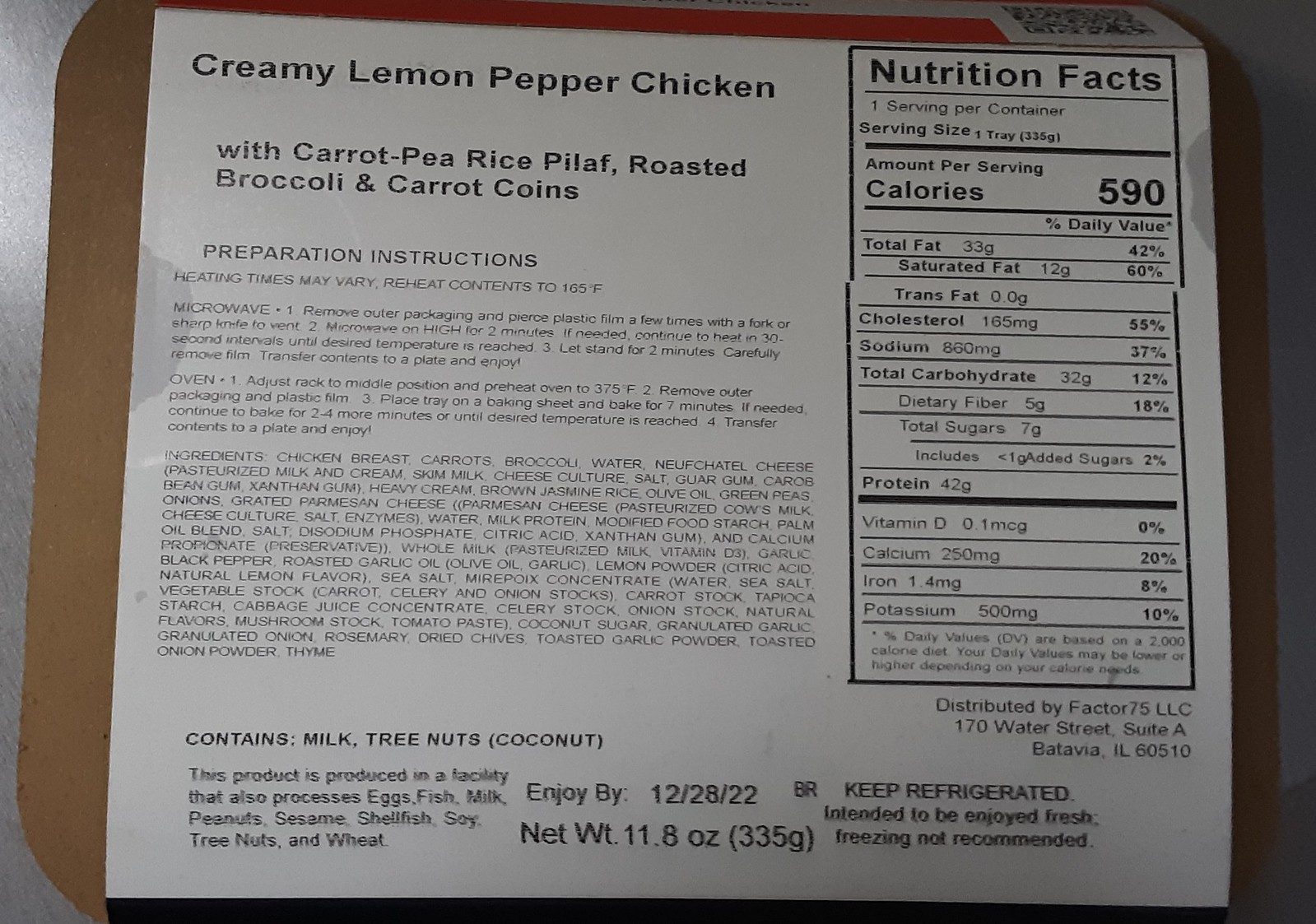This is an image of a packaged TV dinner, specifically labeled as "Creamy Lemon Pepper Chicken with Carrot Pea Rice Pilaf, Roasted Broccoli, and Carrot Coins." The nutritional information provided includes 590 calories, 33 grams of fat, 165 milligrams of cholesterol, 860 milligrams of sodium, 32 grams of carbohydrates, 5 grams of dietary fiber, 7 grams of total sugars, and 42 grams of protein. The packaging also lists detailed ingredients, noting that the meal contains milk, nuts, and coconut. Additionally, both microwave and oven cooking instructions are provided for convenient preparation.